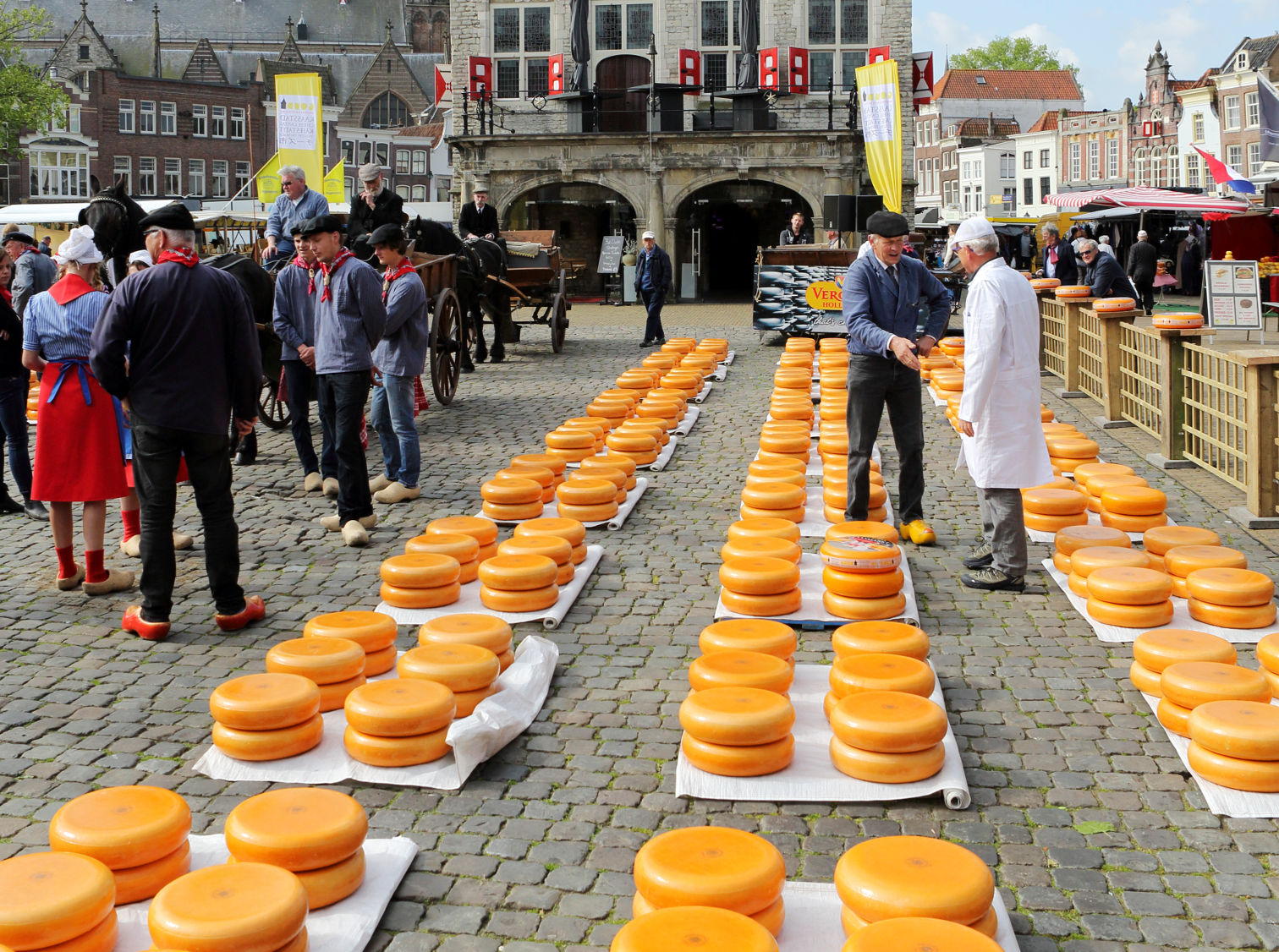The image depicts a bustling cheese market in an old European village, where numerous orange-colored cheese wheels are meticulously arranged on large, white blankets. These cheese wheels are stacked, with many placed two atop each other, forming multiple rows that stretch across the ground. In total, there appear to be three rows, each comprising around eight collections of six stacks. The scene is vibrant, with a man in a long blue sleeve shirt and black pants conversing with a person in a white coat. Among the crowd, men in blue shirts and wooden shoes, as well as a woman wearing a red dress, a red headscarf, and wooden shoes, add to the festive atmosphere. The backdrop features quaint, light stone-colored buildings adorned with red signage that includes white squares, set against a light blue sky flecked with white clouds. Green trees frame the picturesque setting, enhancing the village's charm.